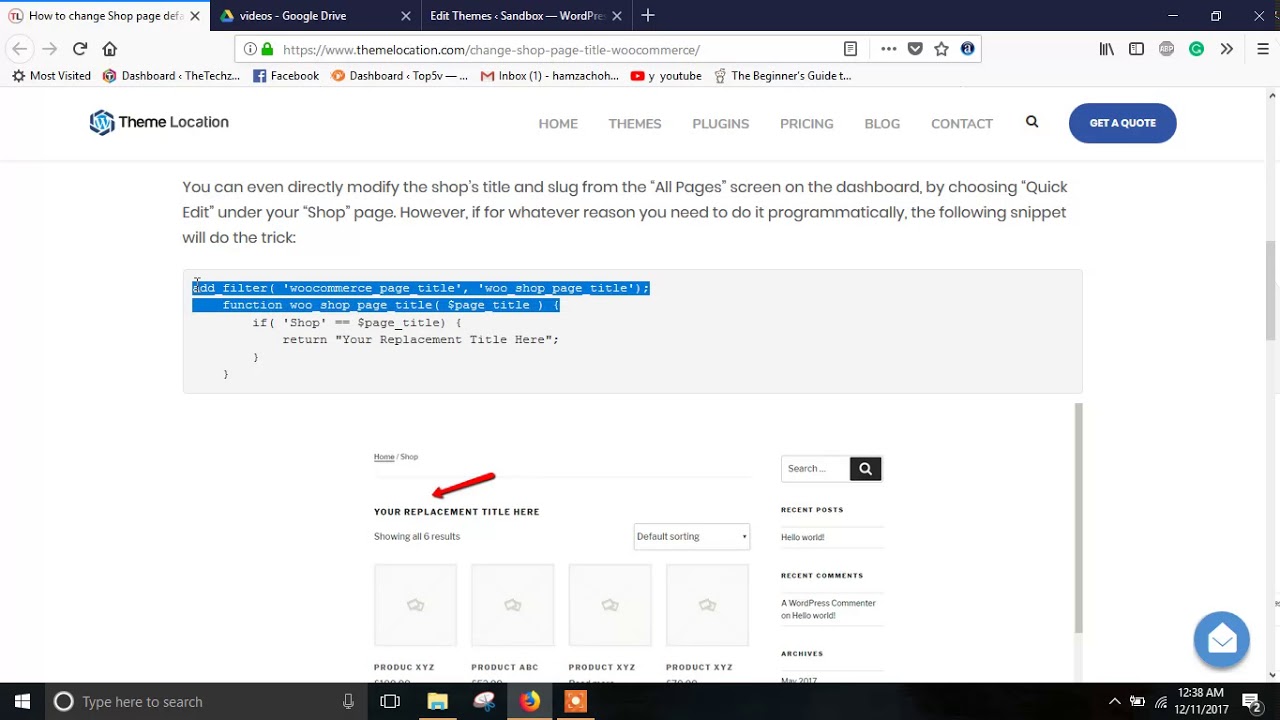Screenshot of a Desktop Computer on a Firefox Browser

The screenshot captures a desktop computer's display, formatted in a wide rectangular shape, with the browser's user interface prominently visible. The browser in use is Firefox, evidenced by the distinctive design elements.

At the top of the browser, a series of tabs are laid out horizontally. The active tab is partially visible, titled "How to Change the Shop Page," though it is cut off. Adjacent tabs include ones labeled as Videos, Google Drive, and Edit Themes, with a plus sign for opening a new tab. In the top right corner, there are the standard system buttons for closing (X), minimizing, and maximizing windows.

The browser's address bar is in the middle top section, containing the standard navigation elements: back and forward buttons, a refresh button, and a home button. Directly below the address bar, a bookmarks bar displays several favorite websites listed as Most Visited, Dash Bears, Dashboard, Facebook, Dashboard Logic, Inbox, YouTube, and Beginner's Guide to.

The main webpage visible in the screenshot showcases a white background and appears to be some sort of editing page with a focus on theme locations. Prominently displayed is a diamond-shaped logo featuring a blue center. The webpage's navigation menu includes links to Home, Themes, Plugins, Pricing, Blog, and Contact, with a gray search button. A blue "Get a Quote" button stands out on the page, and in the upper right corner, there's an icon of an open envelope, likely intended for email contact.

At the bottom of the screen, elements of the Windows operating system are visible, including the taskbar with various icons for time, notifications, and signal strength.

A subtle blur pervades the screenshot, suggesting it is of low resolution, limiting the fine detail that can be discerned. However, the fundamental components and their layout remain identifiable.